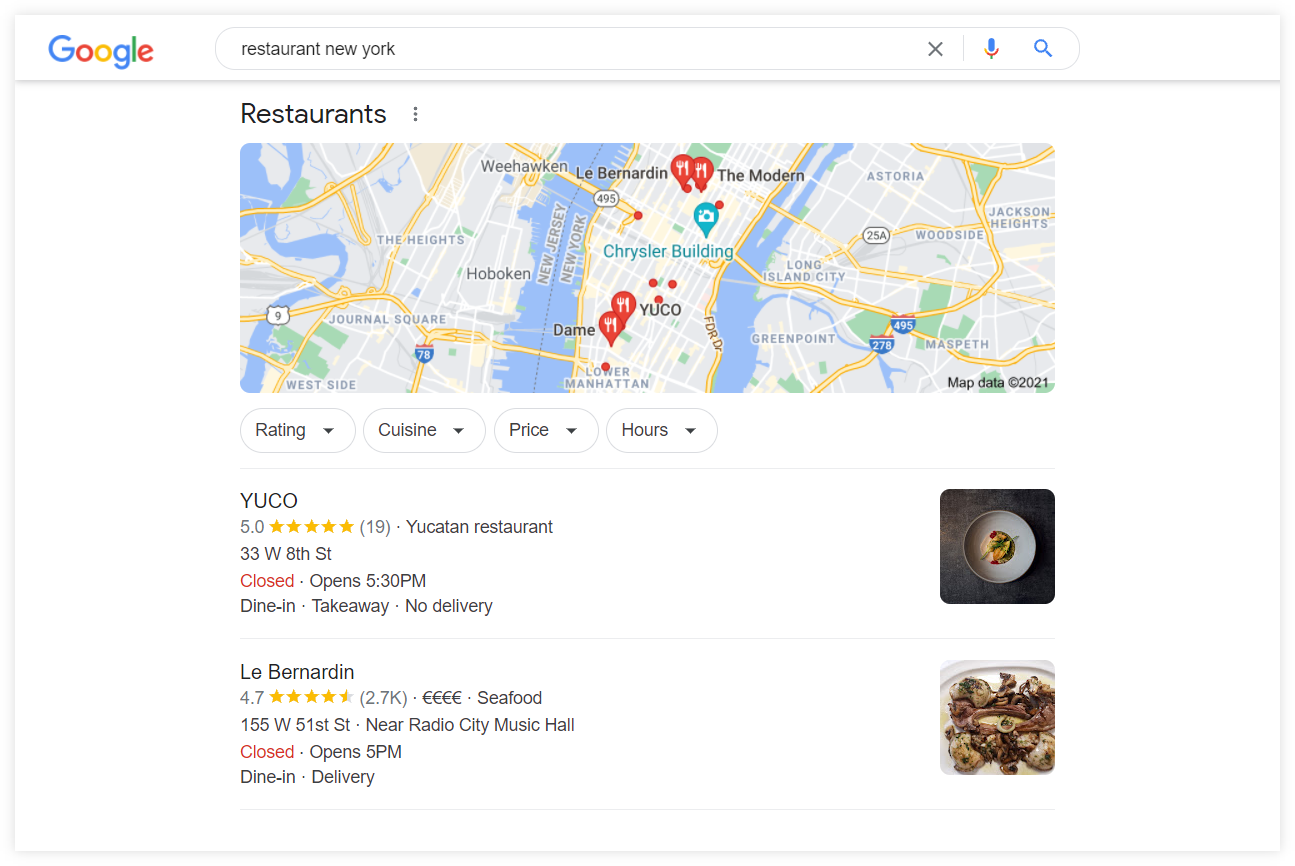In the upper left corner of the image, the Google logo is prominently displayed. To its right, there is a search bar containing the query "Restaurant New York." Adjacent to the search bar are icons: an "X" for clearing the search, a blue microphone for voice input, and a small blue search button.

Below the search bar, the word "Restaurants" appears in bold black text. Dominating the lower portion of the image is a large map, featuring various shades of blue areas, yellow lines representing roads, and prominently displayed in blue text at the center is the label "Chrysler Building." The map also includes interstate signs and multiple red teardrop-shaped markers with a fork and knife icon, signifying the locations of restaurants.

Below the map, the text "YUCO" is displayed in uppercase, accompanied by a five-star rating and the number "19" in parentheses. Next to this, the description "Yucatan Restaurant" is provided, followed by an address: "33 W 8th Street." The text "Closed" is highlighted in red with the note "Opens 5:30 PM" below it. To the right of this information is a black square containing a white circle.

Further below, another restaurant entry is listed: "Le Bernardin," which has a rating of 4.7 out of 5 stars and "2.7K" in parentheses, indicating the number of reviews. To the right of this entry is an image of a plate of food.